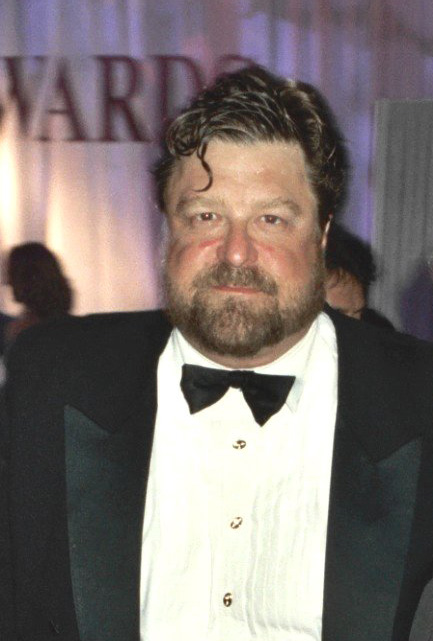In this vintage photograph, John Goodman, recognizable for his role as Roseanne's husband in the television series "Roseanne," stands elegantly in a classic black and white tuxedo. The tuxedo features a traditional penguin style with a black bow tie at the center and distinctive gold buttons adorning the white undershirt, one of which resembles the number six. Goodman's facial hair frames his face, extending from the top of his head down to his chin and upper lip. His short brown hair is slicked back and parted to the side, with a few strands falling across the left side of his forehead from the viewer's perspective. Behind him, a white curtain with partially visible text forms the background, reading "wards" though the full message remains obscured. The backdrop is otherwise blurry, hinting at the presence of a couple of other indistinct figures. The overall composition of the photograph is vertical, emphasizing Goodman's distinguished presence.